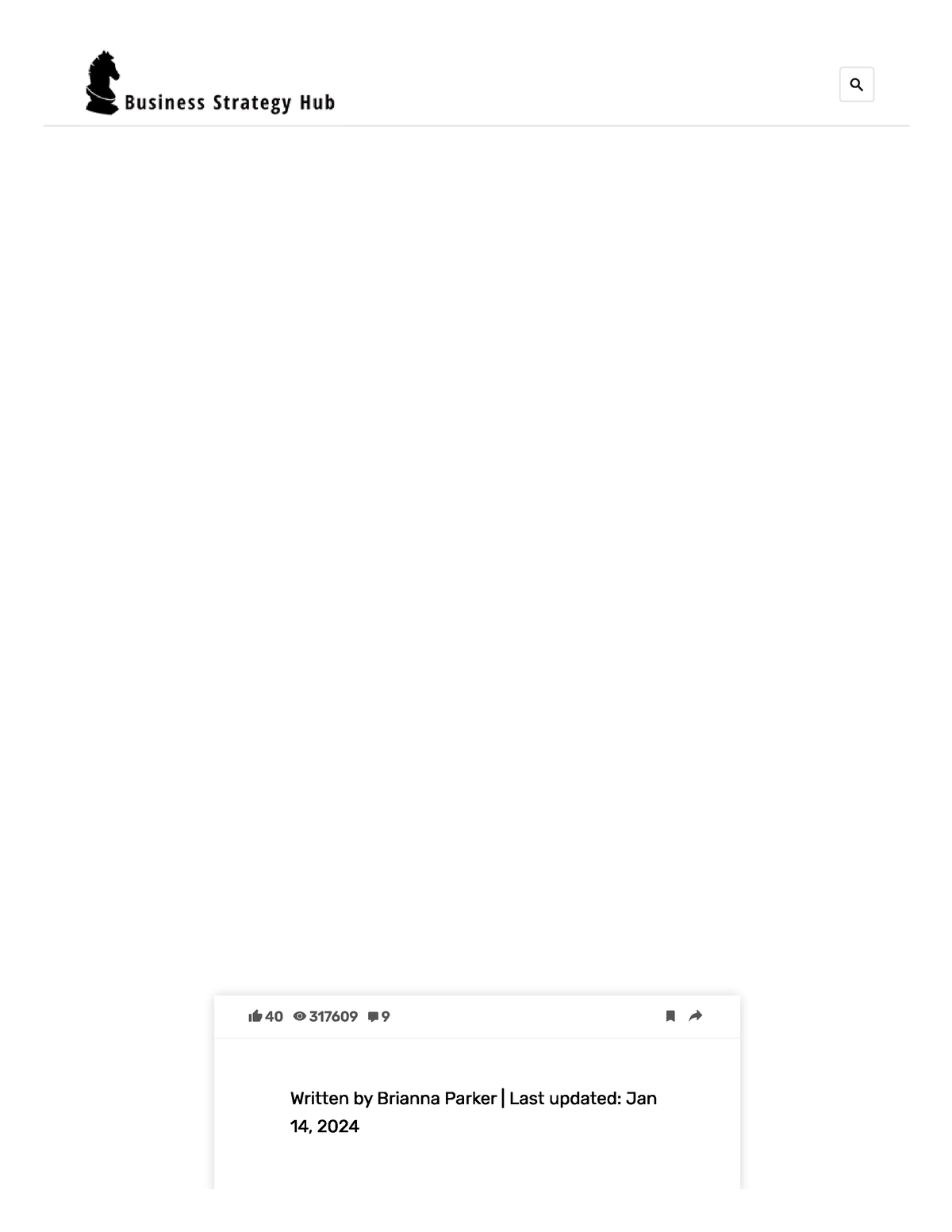The image depicts a minimalistic webpage layout. At the very top, on the upper-left corner, there is a small black chess piece icon. Adjacent to this icon, in very small black letters, is the text "Business Strategy Hub." On the upper-right corner of the page, there's a tiny white square with a small magnifying glass icon, suggesting it functions as a search tool, albeit not in the form of a traditional search bar. A thin gray line runs horizontally under these elements from left to right.

The majority of the screen below this line is completely blank, emphasizing a clean and uncluttered design. At the very bottom of the screen, there's a small rectangle containing several elements. Starting from the upper left of this rectangle, there is a thumbs-up icon followed by the number 40. Next to it, there is an eye icon with the number 317,609, indicating views. A comment bubble icon follows, showing the number 9, representing the number of comments. On the upper right of this rectangle, there's a small square with an arrow pointing outward, suggesting a sharing function. Below this rectangle, it is noted that the content was written by Brianna Parker and last updated on January 14, 2024. This concludes the description of the webpage layout.